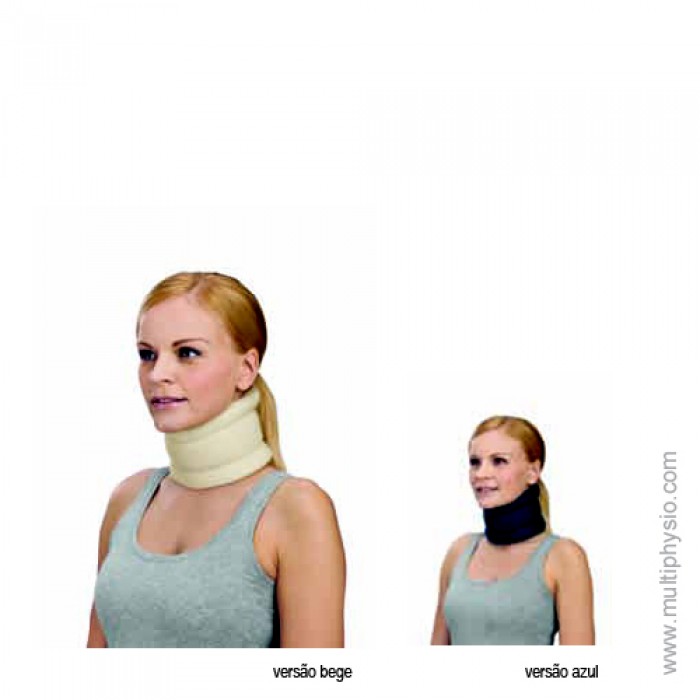The image is a landscape orientation advertisement for neck braces, presented in Portuguese, featuring a red-haired woman with her hair pulled back in a ponytail. The composition consists of two photographs of the same woman in different neck braces and is designed in a photographic representationalism style, combining realism with typography.

On the left side of the image, a larger photograph shows the woman smiling and facing left. She is wearing a gray halter top and a light brown neck brace labeled “Versailles Beige” in black text near the bottom right corner of her elbow.

To the right is a smaller photograph of the same woman in the same attire, this time wearing a dark blue neck brace. The text near the bottom right corner of this photograph reads “Versailles Azul.” Vertically aligned on the right border of the image is the URL “www.multiphysio.com” in gray type.

The overall advertisement prominently displays the neck braces while ensuring brand visibility and maintaining a clean, professional aesthetic.